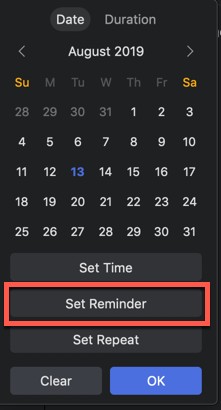This image captures a slightly tilted, off-center photograph of a reminder-setting menu, suggesting it wasn't taken as a direct screenshot. The interface seems to be in dark mode, featuring a carbon-colored background with muted, matte-textured elements. Displayed prominently is a calendar set to August 2019, with the 13th selected. The menu includes "Date" and "Duration" options, with "Date" currently active. Situated below these options are three buttons: "Set Time," "Set Reminder," and "Set Repeat," with "Set Reminder" highlighted in a red box. At the bottom, there are "Clear" and "OK" buttons, presumably to reset or confirm the reminder settings. Despite the detailed illumination of the menu options, there is no indication of the current date.